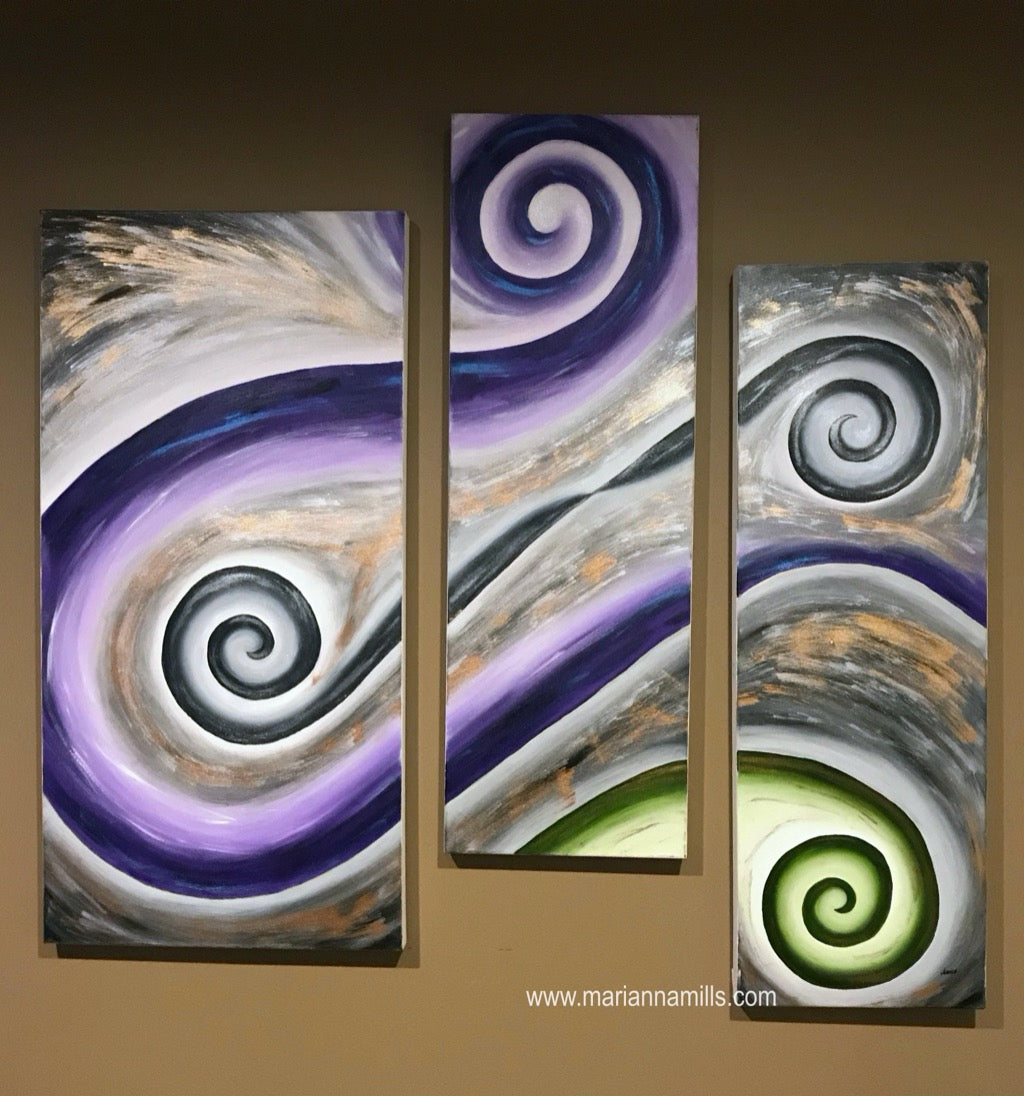This image showcases an abstract three-piece art installation, prominently displayed on a wall, potentially in a gallery or home setting. The installation features three rectangular canvases of varying sizes and dimensions, arranged in an intentionally jagged, non-parallel manner. The left panel is a rectangular white board, with the middle panel being narrower and positioned slightly higher. The third, and largest panel, resides on the right side, set a bit lower. Together, these panels converge to create a cohesive design. The artwork within these panels presents a mesmerizing array of swirling patterns and loops, primarily using hues of purple, lavender, white, black, green, and occasional bursts of orange and tan. The intricate loops, resembling graceful snakes, intertwine and curl upon themselves, creating a dynamic wave-like effect across the canvases. Additionally, a watermark reading "www.marianamills.com" is present at the bottom of the artwork, identifying the piece's origins.